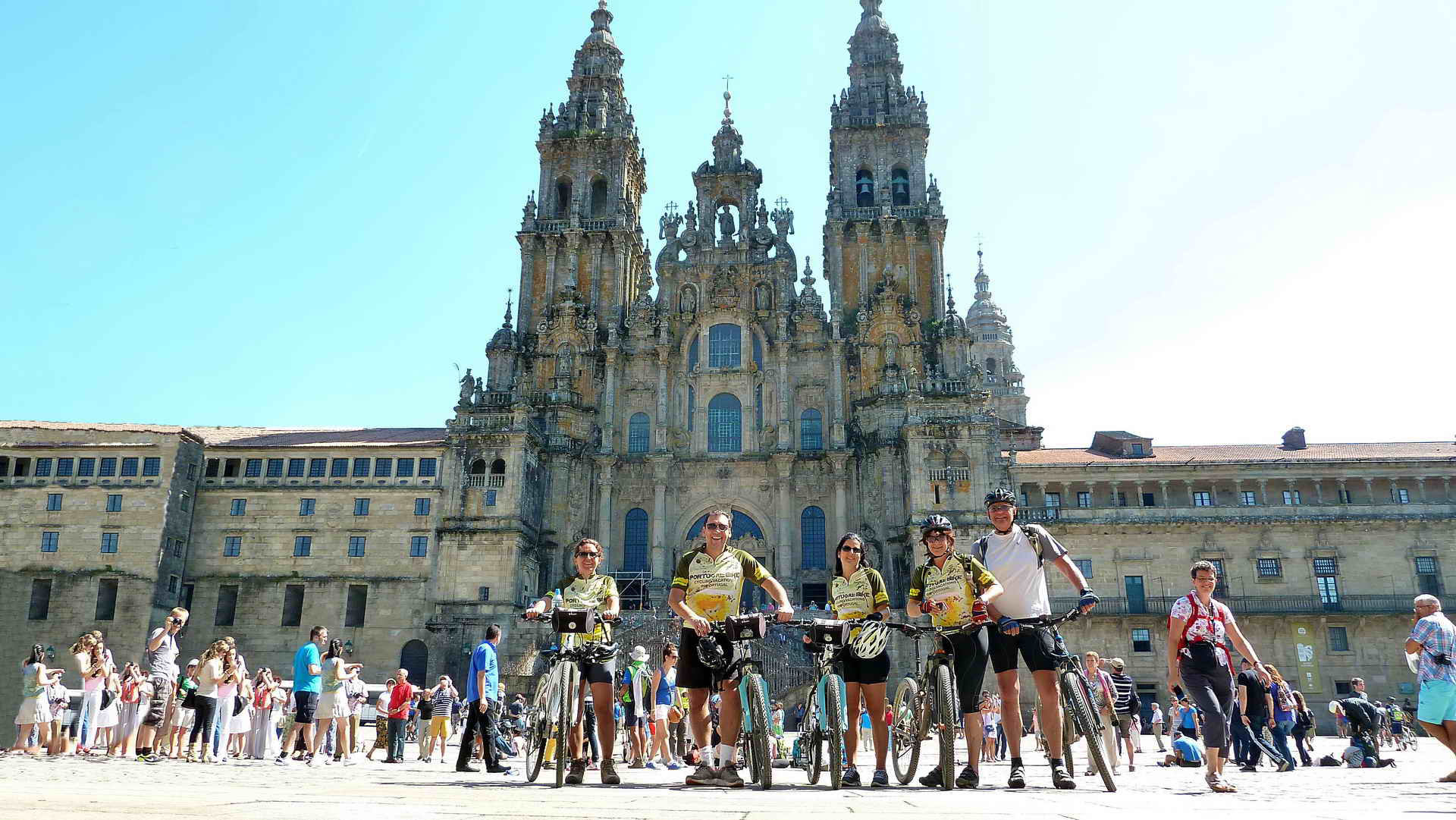In this vibrant photograph, a group of five cyclists stands proudly next to their bicycles, all facing the camera with determined expressions. Four of them are clad in matching yellow and black uniforms, while the person on the far right stands out in a white shirt and black shorts. This individual, along with the girl beside him, are both wearing helmets and sunglasses, beaming with smiles. Behind the group, a crowd of onlookers adds to the bustling atmosphere. Dominating the background is an impressive, ornate cathedral with two towering spires flanking a slightly shorter central section, adorned with intricate pillars. Adjacent to the cathedral are several multi-story stone buildings, each featuring numerous windows. The scene is bathed in sunlight, under a clear blue sky, capturing the essence of a perfect sunny day.